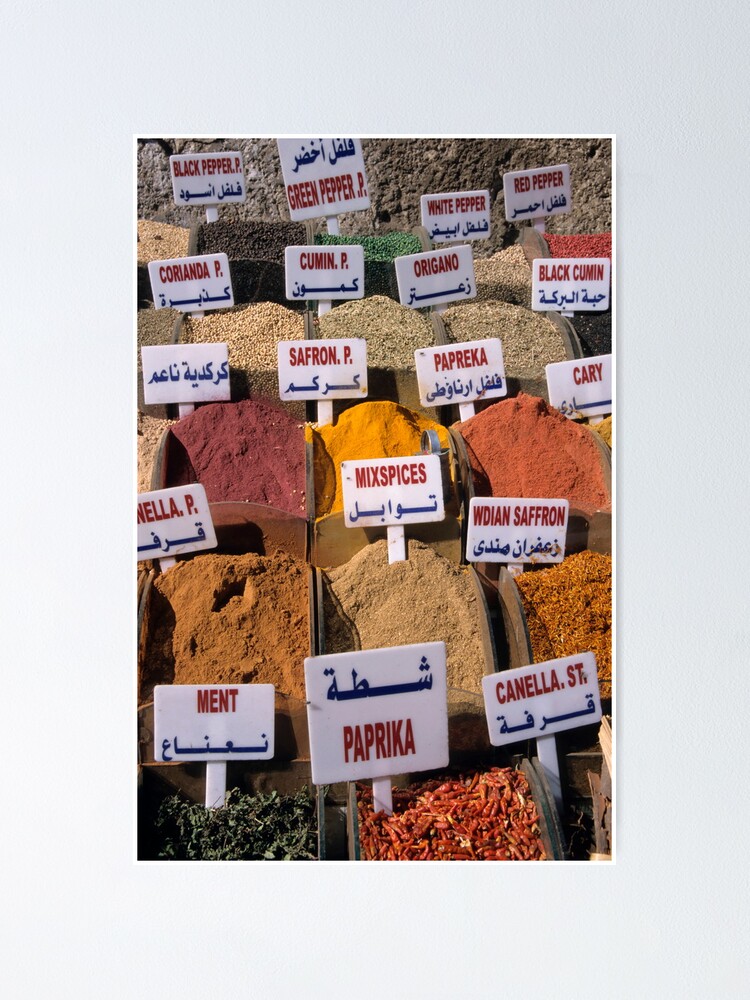This photo captures a vibrant market scene, likely set in a Middle Eastern country, showcasing a diverse array of spices. The spices, arranged in numerous bins on a shop table, include black pepper, green pepper, white pepper, black cumin, curry, Indian saffron, saffron pea, paprika, mixed spices, canola, oregano, coriander, and mint. Each spice bin is labeled with signs in both English and Arabic, although some signs have minor misspellings (e.g., "M-E-N-T" instead of mint). The spices are displayed in large quantities within wooden containers approximately four by six inches in size, suggesting that customers can scoop out and purchase significant amounts, such as up to half a pound. The rich colors and varied textures of the spices, ranging from the emerald green of mint to the deep red of paprika, create an exciting and visually stimulating scene.